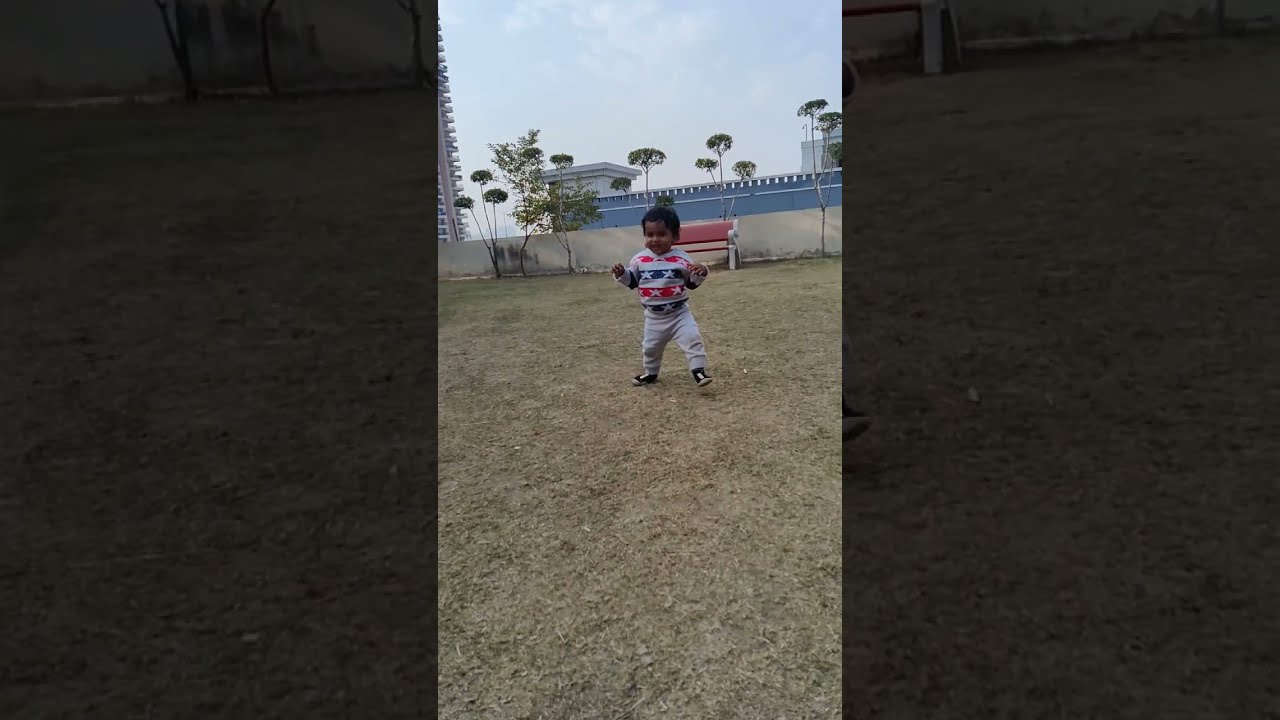The image captures a Hispanic toddler, possibly around two years old, with dark brown or black hair, stepping towards the camera. The child is dressed in a gray long-sleeve shirt with red and blue stripes or bars, featuring images of turtles or dinosaurs, and is paired with gray sweatpants and blue sneakers. The setting appears to be a park or a dry, grassy field within a city, suggested by the presence of a tall apartment building and other large buildings in the background. Behind the child, there is a distinctive red bench with white handrails and several newly planted, trimmed trees growing near a concrete wall. The sky above is blue with some white clouds, indicating this scene takes place during the daytime.